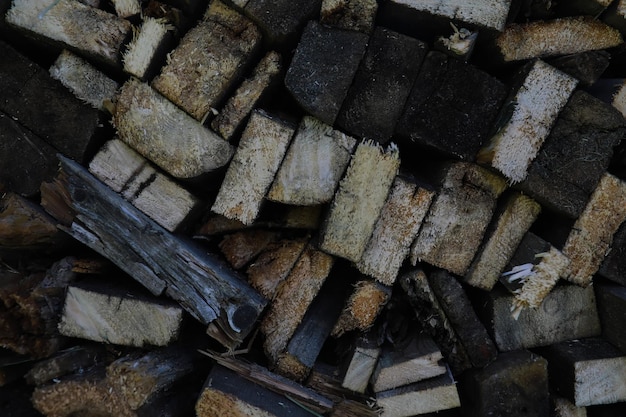The photograph showcases a cluttered pile of chopped wood blocks, turned to display their rough, freshly cut faces. The diverse assortment includes pieces of varying colors and conditions — some light and fresh, others darkened, charred, or dirty. The exposed grains and textures reveal further details, with some blocks appearing damp or waterlogged while others seem dusty. A few blocks stand vertically, accentuating their jagged edges and cuts, while others lie horizontally, revealing more grooves and cracks. The dim lighting enhances the textural contrasts and the natural imperfections of the wood, giving the image a rustic, almost artistic quality. Scattered wood chips add to the chaotic yet intriguing arrangement, emphasizing the varied and naturally flawed aesthetic of the scene.